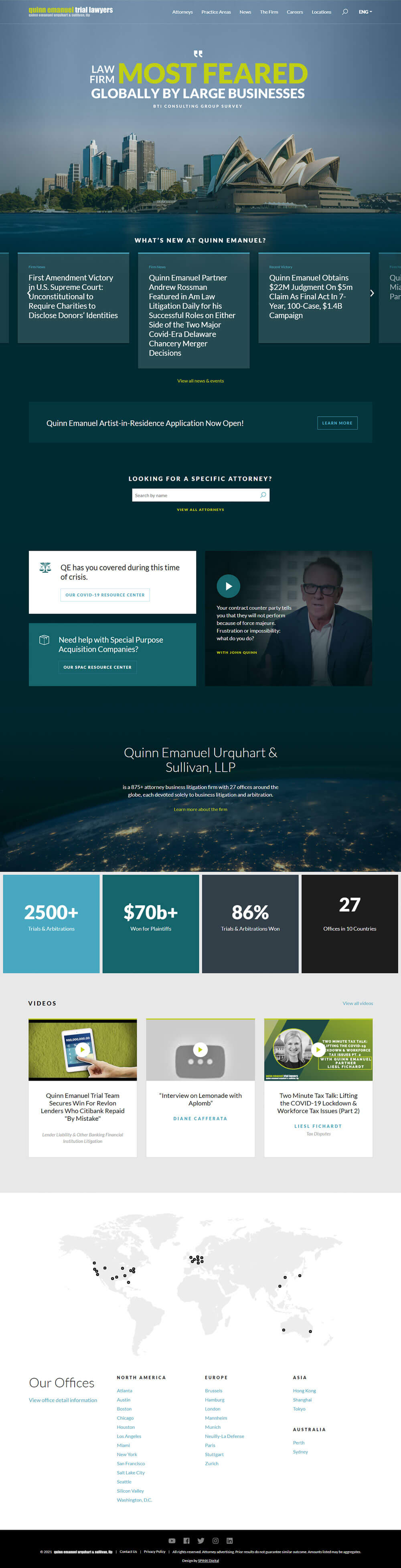The image portrays a webpage from Quinn Emanuel Trial Lawyers, titled "Law Firm Most Feared Globally by Large Businesses," based on a BTI Consulting Group Survey. The top section of the webpage includes navigation links for various categories such as Attorneys, Practice Areas, News, The Firm, Careers, Locations, and a search icon represented by a white magnifying glass.

Prominently displayed is the firm's name, Quinn Emanuel Trial Lawyers, followed by a section titled "What's New at Quinn Emanuel?" This section features multiple headlines, including:

- "First Amendment Victory in U.S. Supreme Court: Unconstitutional to Require Charities to Disclose Donors' Identities."
- "Quinn Emanuel Partner Andrew Roseman Featured in A.M. Law Litigation Daily for His Successful Roles on Either Side of the Two Major COVID-Era Delaware Cancer Merger Decisions."
- "Quinn Emanuel Obtains $22 Million Judgment on $5 Million Claim as Final Act in 7-Year, 100-Case, $1.4 Billion Campaign."

A "View All News and Events" button invites users to explore further. Additionally, the page announces that "Quinn Emanuel Artist in Residence Applications Now Open," accompanied by a blue "Learn More" button.

A search field allows visitors to look up specific attorneys by name. The page also includes various images and statistics highlighting the firm's achievements.

At the bottom of the webpage, there's a detailed map marking Quinn Emanuel's office locations in the United States, Europe, Asia, and Australia, with dots indicating these global offices.